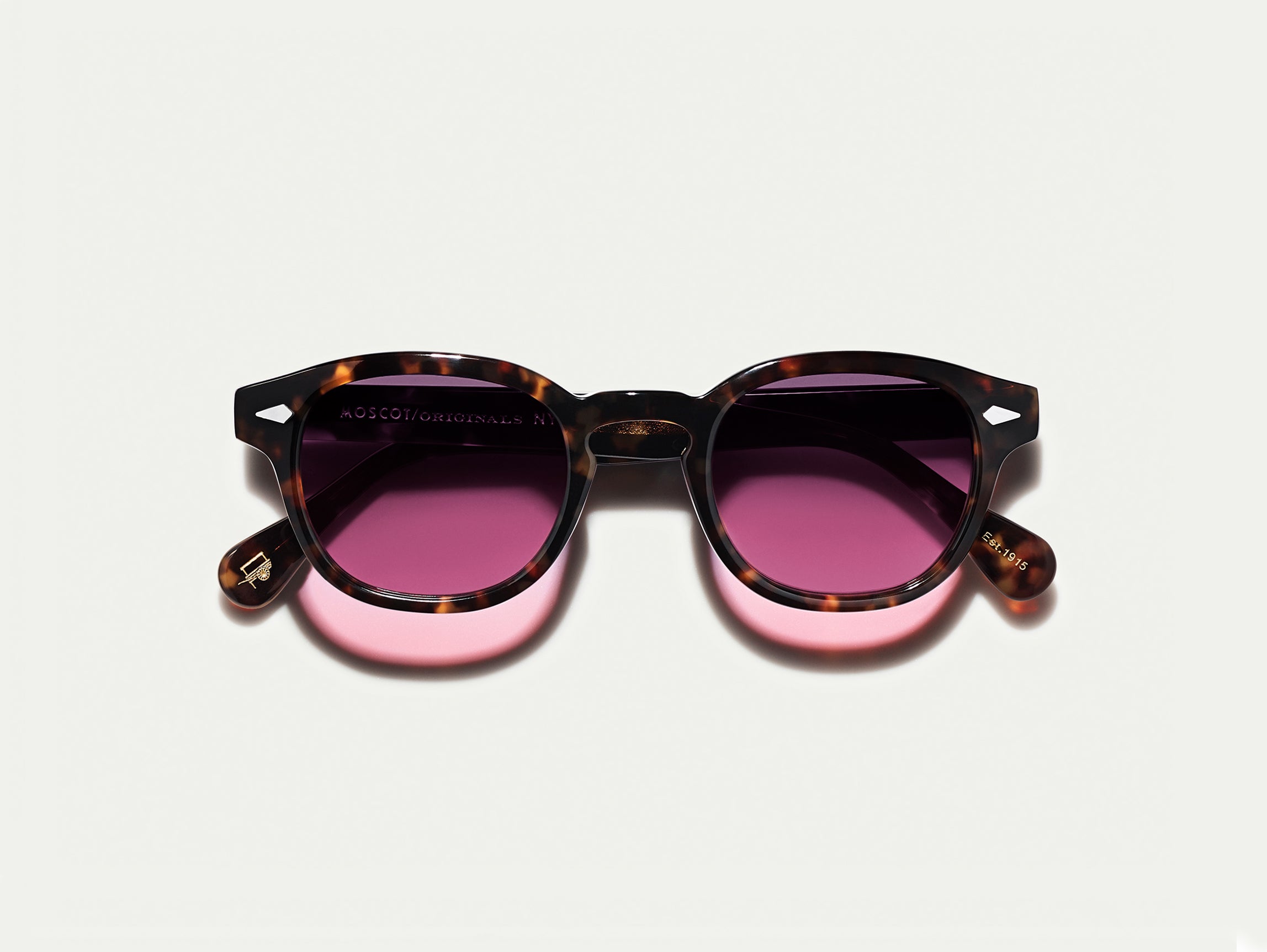The image showcases a pair of women's fashion sunglasses resting on a plain white background. The sunglasses have a distinctive tiger print frame, blending shades of brown and orange, with a slightly rounded shape that is not entirely circular nor cat-eye. Notably, there is a silver dot accent by each eye and hinge, adding a touch of elegance to the design. The lenses are rose-colored with a purplish, almost plum hue, casting a pinkish shadow on the white surface beneath them. Although some writing and a possible logo are present on the earpieces, the details are not readable. The frames are made of plastic, and the sunglasses are folded flat with the earpieces down, emphasizing their compact form. These trendy sunglasses likely appeal to a younger audience, given their stylish design and vibrant lens color.